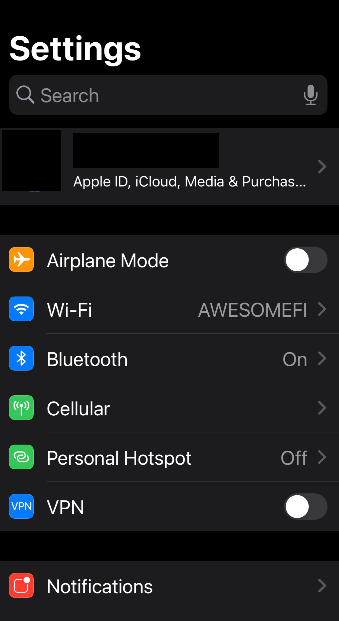The image displays a screenshot of the Settings menu on a smartphone with a black background. At the top-left corner, the word "Settings" is prominently displayed in large white letters. Below this, a dark gray banner contains a light gray search icon with the word "Search" in gray text, and a gray microphone icon on the far right.

Further down, another dark gray banner shows a black square and a black rectangle on the left, followed by the text "Apple ID, iCloud, Media, and P-U-R-C-H-A-S…" in white, and a gray arrow pointing to the right.

Below this banner, the screen is divided into sections each marked by dark gray backgrounds. The first section begins with "Airplane Mode" written in white, accompanied by an orange square featuring a white airplane icon. A toggle button on the right is white and positioned to the left, indicating that Airplane Mode is off.

The next item is "Wi-Fi," labeled in white text. It features a blue box with a white Wi-Fi icon, and the name "Awesome Fi" on the right with a gray arrow indicating navigability. Below this, a thin gray line separates the entries.

Following is "Bluetooth," displayed with a blue box and a white Bluetooth icon. It is marked as "On" in gray text to the right, alongside a gray arrow.

Next is "Cellular," indicated by white letters and a green box with a white cellular signal icon. It has a gray arrow pointing to the right. 

Afterward, "Personal Hotspot" is shown with a green square containing two linked white ovals, and it reads "Off" to the right with another gray arrow.

Lastly, "VPN" is depicted with a blue square and white text, including a white VPN icon. Its toggle switch is white and positioned to the left, showing that the VPN is off.

At the bottom section, the screen displays "Notifications" in white text. This is featured on a dark gray background with a red square, containing a white box with a small white circle inside it, and a gray arrow pointing to the right.